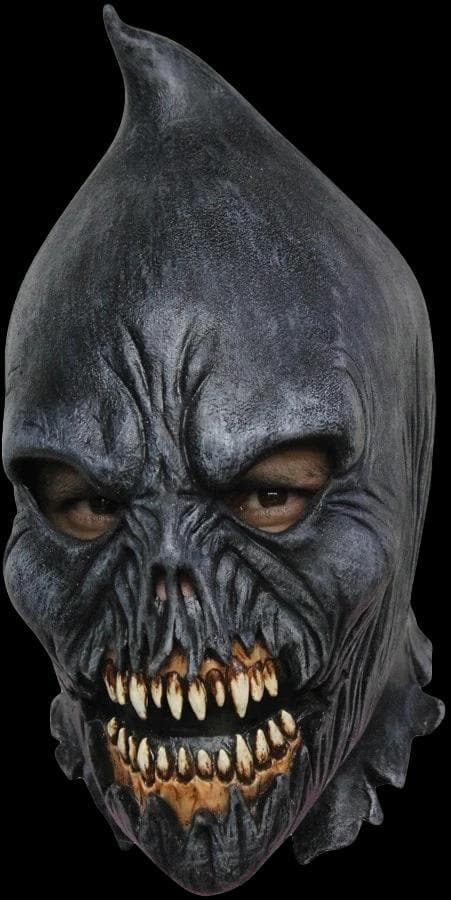The image depicts a man wearing a terrifying black leather face mask that conjures the visage of a demonic, ghostly creature. The mask is pointed at the top and closely fits over the head, hiding the ears and forming deep folds of textured leather around the forehead. The eye openings are shaped, revealing the man's eyes beneath. The nostrils are represented by two jagged holes, surrounded by wrinkled leather, leading down to high, sharp cheekbones. The most menacing feature is the mouth: ripped open in a perpetual roar, exposing long, sharp fangs. The gums are yellow near the top, transitioning into brown roots, and the teeth are a stark ivory at the edges. The interior of the mouth is entirely black, enhancing the eerie effect. The chin tapers to a point, and the mask extends fully down over the wearer’s chin. The photo, set against a black background, captures the full extent of the mask's ferocity and dark design.